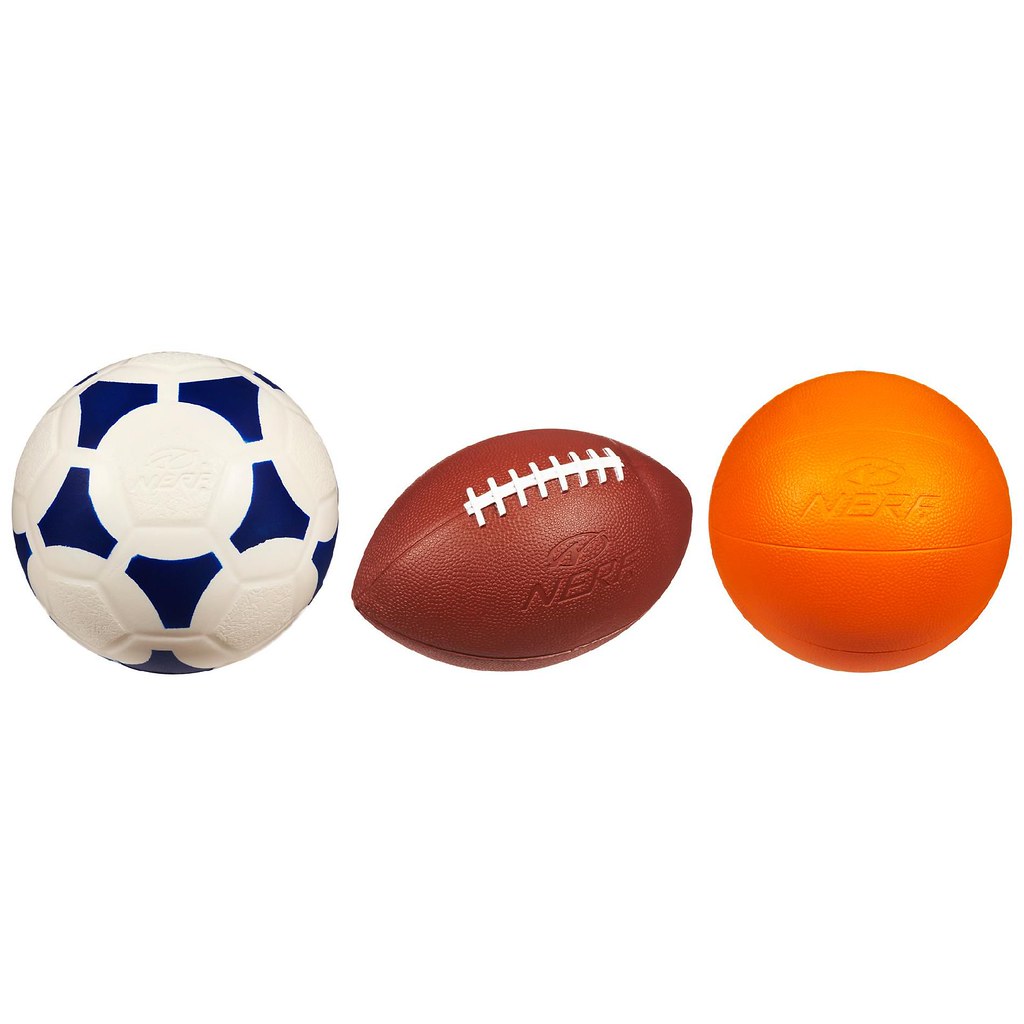The image displays three Nerf sports balls aligned in a row against a pristine white background. From left to right, the balls are a soccer ball, a football, and a basketball. 

The soccer ball on the left is predominantly white with navy blue patterns, resembling a gear or star with a circular design in the center. The ball features the Nerf logo in white, blending seamlessly with its surface.

In the middle, the football is brown with prominent white laces and hand grips. The Nerf branding is also in brown, subtly blending into the ball's surface. This football is clearly modeled after an American football.

The ball on the far right is an orange basketball, complete with textured dots for grip. It sports the Nerf logo in orange, matching its overall color. 

All three balls appear to be made out of Nerf's characteristic foam material, making them squishy and safe for indoor play. The white background accentuates the vibrant colors and designs of the balls, bringing them into sharp focus.